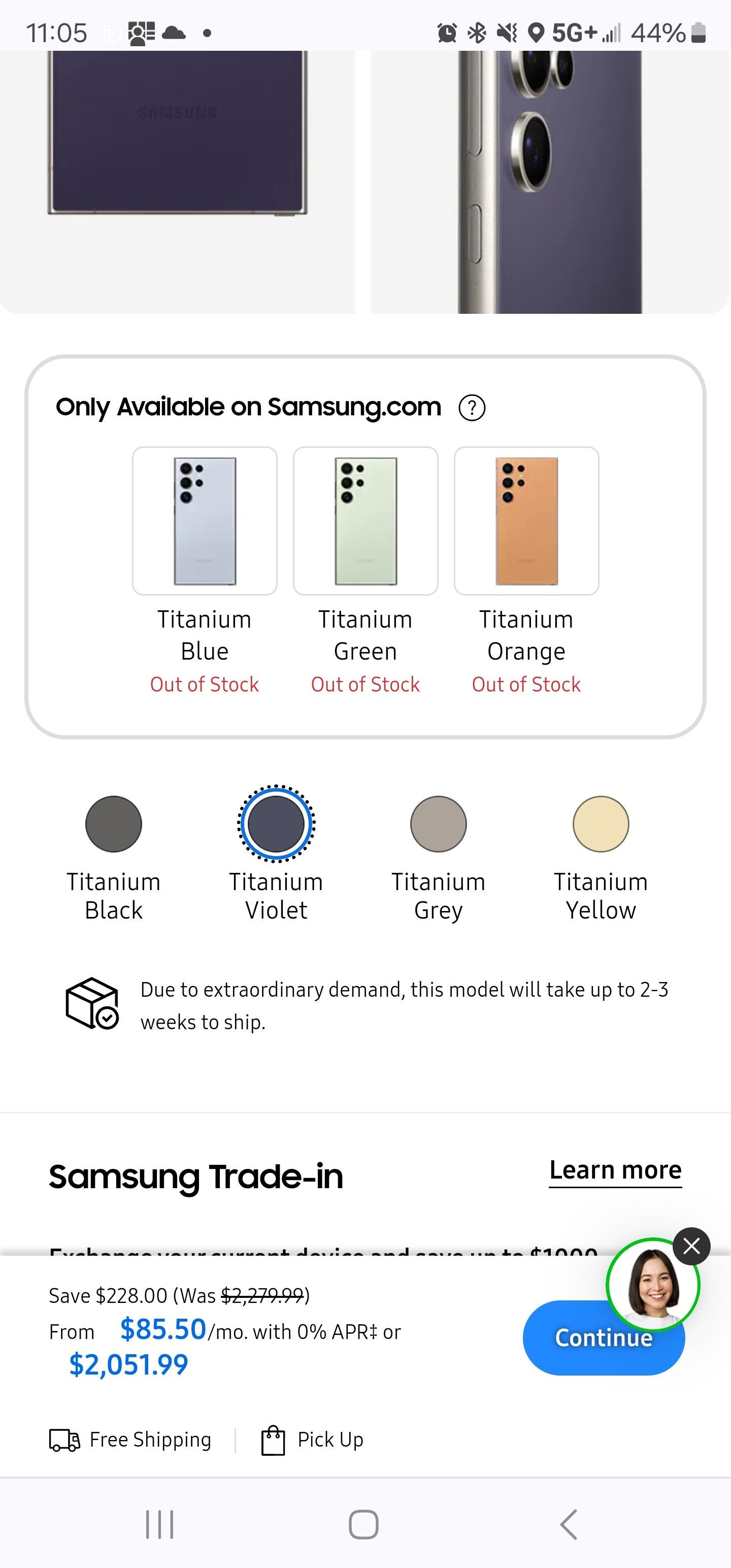The screenshot captures the online shopping experience on Samsung's website for a cell phone. At the top of the screen, the status bar indicates the time as 11:05, with an active alarm set and the Bluetooth connected (currently at 44%). The device is on a 5G+ network with a weak signal.

Prominently displayed are two square images of the phone: the left image shows the bottom back of the device, while the right image highlights the top back, including the camera setup. Below these images, a note specifies that the phone is only available on Samsung.com, accompanied by a clickable question mark for more information.

The phone is shown in three colors: Titanium Blue, Titanium Green, and Titanium Orange, each labeled as "Out of Stock" in red. Additional color options listed below include Titanium Black, Titanium Violet, Titanium Gray, and Titanium Yellow. A disclaimer indicates that due to extraordinary demand, shipping may take up to two to three weeks.

Further down, there's a mention of Samsung Trade-In with a "Learn More" hyperlink. A popup at the bottom announces a savings offer of $228, indicating the original price was $2,279.99, now available for $2,051.99 or $85.50 per month with zero APR. A blue "Continue" button is provided for proceeding with the purchase. Additionally, a floating image of a woman's head suggests availability for live text chat with customer support.

At the very bottom, the notice guarantees free shipping and pickup for the order.